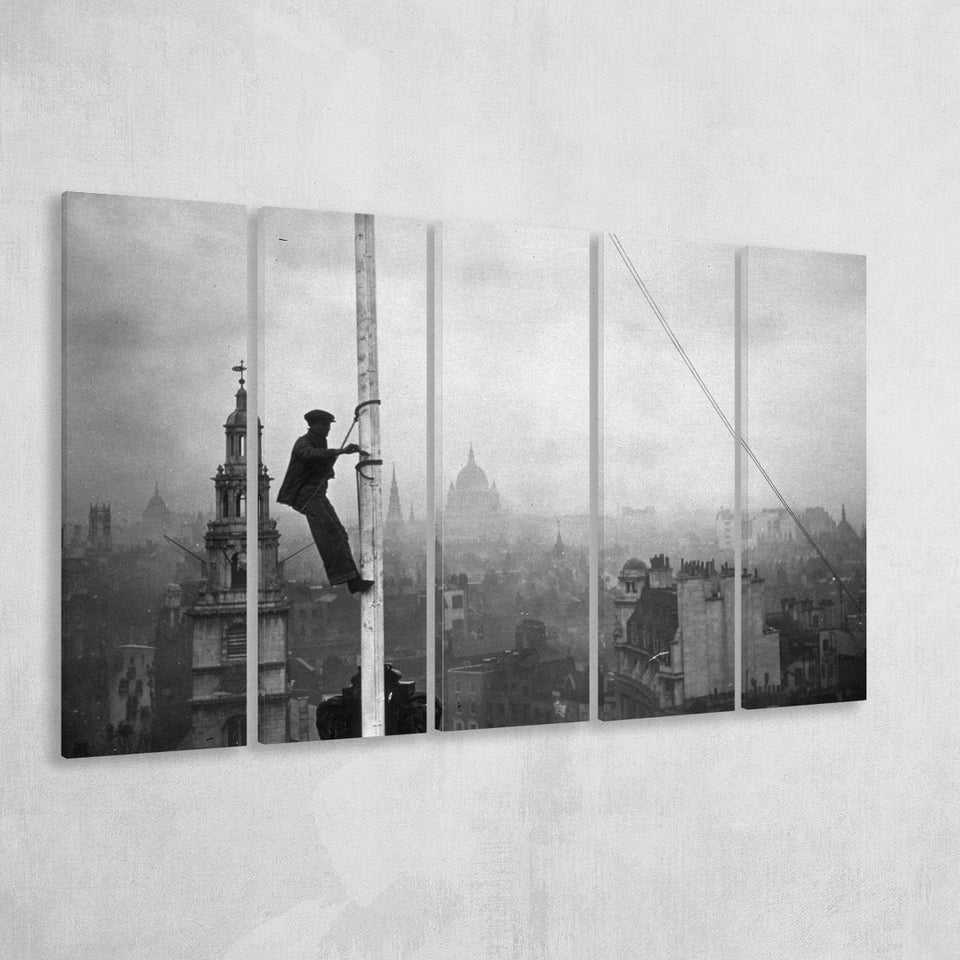This artwork features a striking black-and-white photograph divided across multiple thin, rectangular canvases, which are slightly spaced apart to form one cohesive image. The scene depicts an older, industrial-era European cityscape, possibly from the late 19th or early 20th century, laden with iconic cathedrals, domes, and gothic structures. Against this historic backdrop, a man—likely a construction worker or electrical worker—climbs a large, cylindrical pole. He is adorned in period attire, including wide-leg trousers, a jacket, and a distinctive flat cap or bowler hat. His precarious position halfway up the pole is secured by two ropes wrapped around his head and waist. The background reveals a smoky or foggy haze, enhancing the aged and industrious atmosphere of the city. The artwork, presented on five separate canvases, collectively captures the essence of a bygone era, evoking a sense of both architectural grandeur and the rugged labor that shaped it.